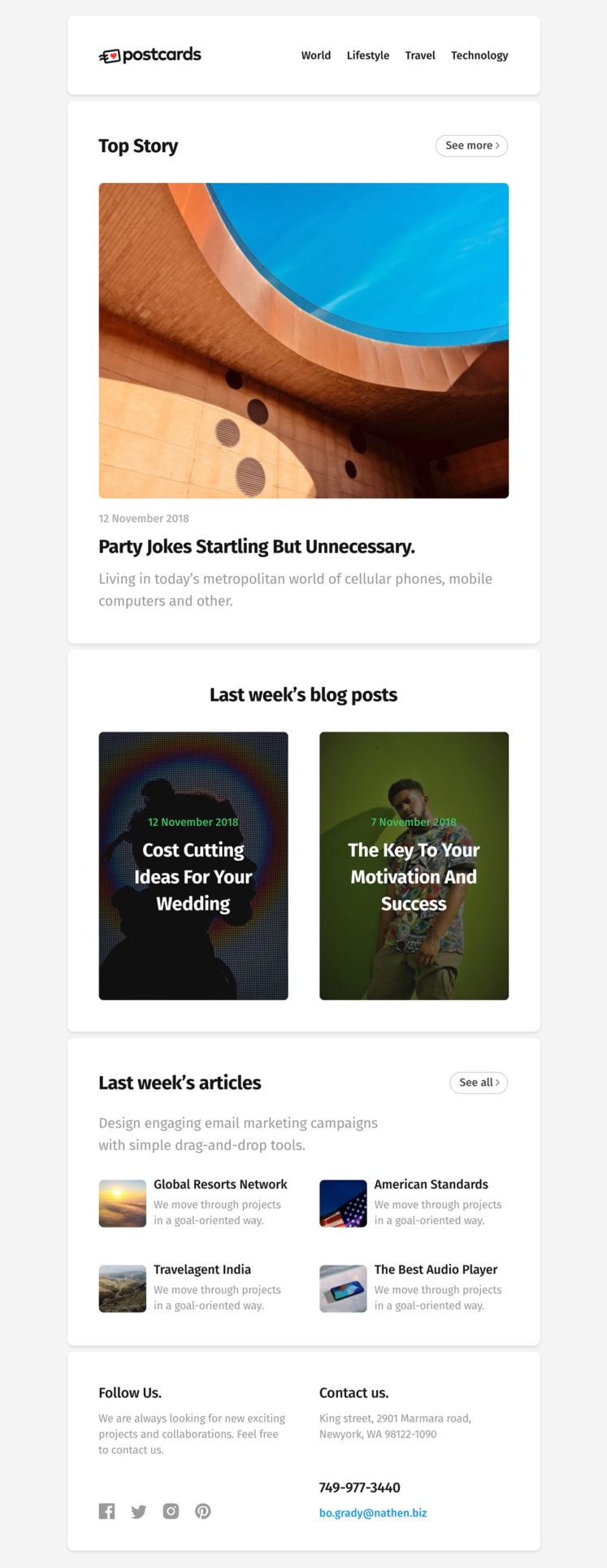Here is a detailed and cleaned-up descriptive caption for the image:

---

The image is a screenshot of a website's homepage, showcasing various sections and navigation options. At the very top left, the word "Postcards" is prominently displayed, followed by navigation tabs labeled "World," "Lifestyle," "Travel," and "Technology" towards the right.

The main image of the page features a circular blue window set against a backdrop of wood, adding an element of rustic charm. In the upper left corner of this image, "Top Story" is written, and below it, the somewhat garbled text "Party jokes starting but unnecessary" appears.

Underneath the main image, there is a section titled "Last Week's Blog Post," which contains two square thumbnails. The first thumbnail is labeled "Cost Cutting Ideas for Your Wedding," and the second one is titled "The Key to Your Motivation and Success."

Further down, another section is labeled "Last Week's Articles," featuring four articles: "Global Resorts Network," "Travel Agent India," "American Standards," and "The Best Audio Player."

At the very bottom of the page, two sections are displayed side-by-side. The left section titled "Follow Us" features icons for Facebook, Twitter, and YouTube, each providing clickable links to those sites. The right section titled "Contact Us" provides a phone number and an email address, offering avenues for direct communication.

---

This caption effectively describes the webpage's layout and content, providing a clear and comprehensive overview.